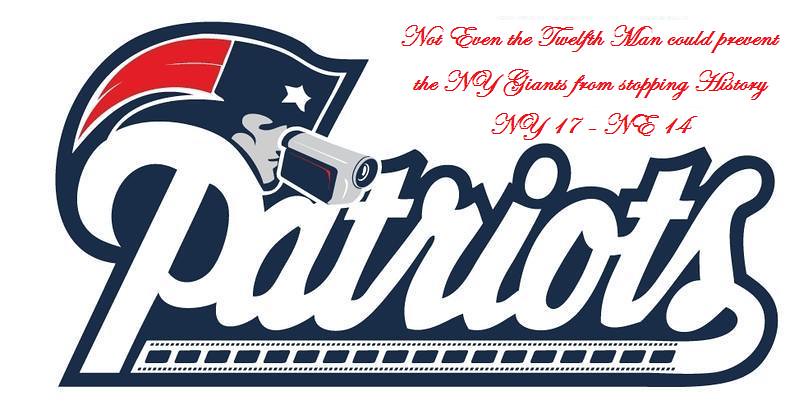In this image, the main focus is the logo of the New England Patriots from the NFL, positioned in the top left corner. The logo features the head of a Revolutionary War-era character with a camcorder around its eye, making a tongue-in-cheek reference to the Spygate controversy. The character has long red hair, with a blue section displaying a white star. At the top right of the image, red text written in a calligraphy-like style states, "Not even the 12th man could prevent the New York Giants from stopping history. New York 17, New England 14." The bottom half of the image boldly displays the word "Patriots" in blue and white ink, adding to the overall tribute style commemorating the Giants' Super Bowl victory over the Patriots. The background is further enhanced by the presence of something resembling a film strip below the Patriots logo.